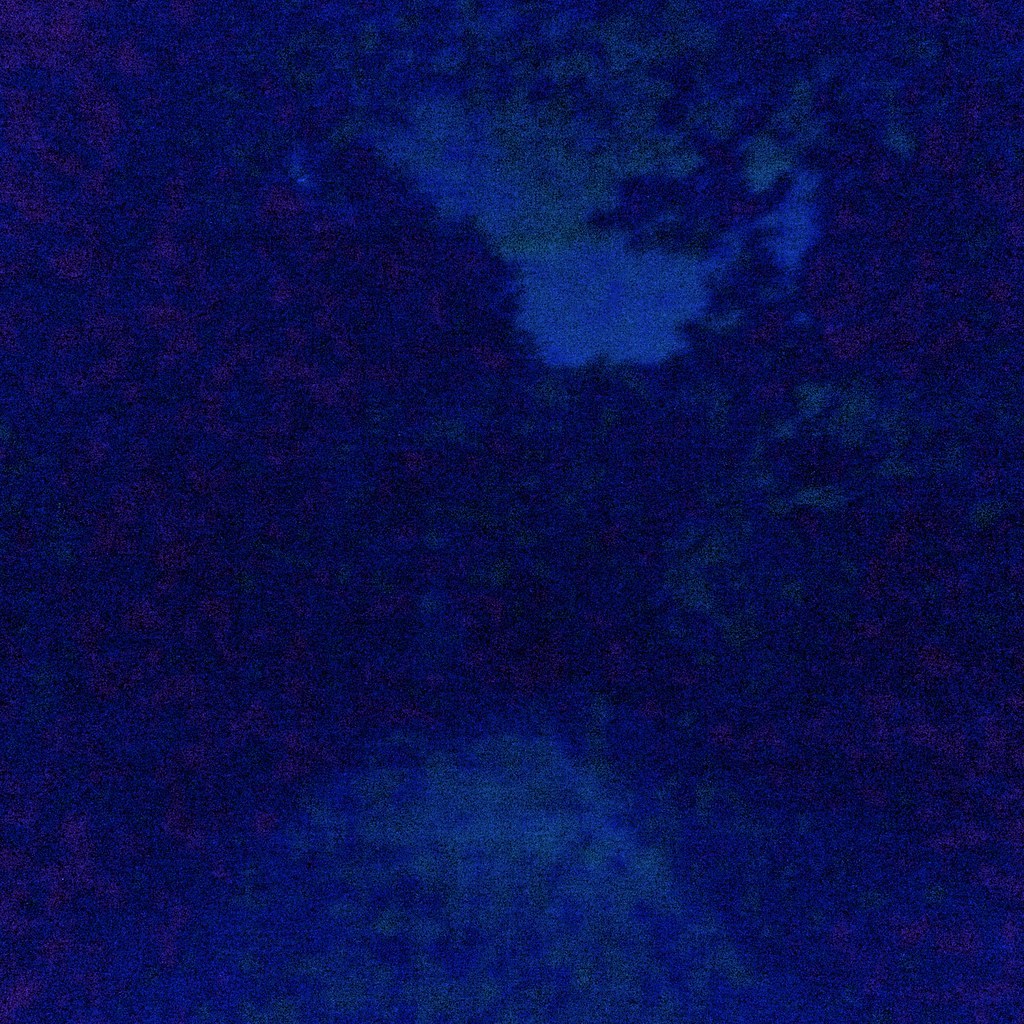This photograph, enveloped entirely in shades of blue, exudes a mysterious, dreamlike atmosphere likely captured during the night or in low light conditions. The image is somewhat blurry, enhancing the ethereal quality and adding to the uncertainty of the scene. At the bottom of the photograph, there is a lighter blue area indicating a narrow lane or path meandering into the distance. Flanking this path, various trees and bushes emerge, their forms softened and somewhat indistinct. Above, the upper section of the photograph showcases a patch of lighter blue, suggesting a glimpse of the sky. The treetops and foliage appear in diverse shapes with hints of what seems to be green, providing subtle yet crucial splashes of color amidst the dominant blue hues. This poignant composition evokes the feel of a nocturnal stroll through a secluded, wooded path under a serene sky.